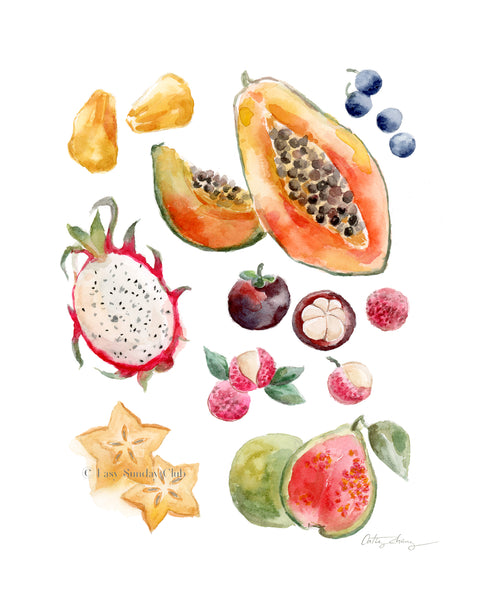This detailed watercolor illustration showcases a vibrant array of fruits set against a plain white background. Prominently featured in the center is a large papaya accompanied by a slice, revealing its vivid orange interior. Above the papaya are several small blueberries. To the left of those is a cut-open dragon fruit, displaying its speckled core. Below the papaya are a couple of lychees, their white insides contrasting with their rough exteriors. In the upper left corner, a cluster of what appears to be chunky pineapple pieces can be seen, while to the right of them, a guava adds a touch of soft green. The lower left corner of the illustration features two delicately-rendered star fruit slices, their unique shape and texture meticulously detailed. There's a signature at the bottom, albeit it's very light and small, nearly blending into the background. A watermark reading "Easy Sunday Club" subtly overlays a part of the artwork, ensuring the artwork's authenticity. The vibrant layers and depth of each fruit suggest a careful application of glaze, bringing a rich, lifelike quality to the illustration.